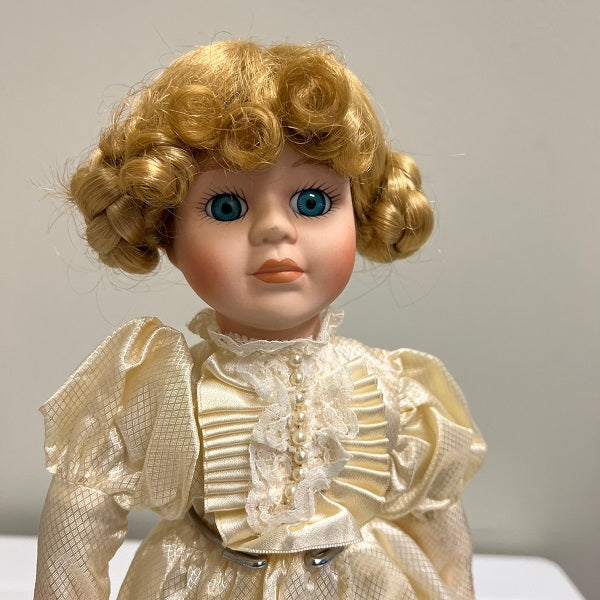The photograph features a detailed porcelain doll dressed in a luxurious, ornate gown that appears to be an elegant blend of cream and pale gold silk. The gown is adorned with intricate patterns and criss-crosses that create a diamond effect, and it is further embellished with pearls meticulously placed in a straight vertical line on a Chantilly lace overlay. The shoulders of the dress have a delicate lacy effect overlaying the cream satin fabric.

The doll herself has a captivating appearance with golden blonde hair styled into tight curls, braided and bunched up around her ears. Her face is delicately painted with rosy blush, neutral pink lips, and striking blue eyes with long, dramatic eyelashes and strawberry blonde eyebrows. She has a slightly somber expression, adding to her antique charm.

The doll is positioned on a white table against a plain white background, supported by a metal hook around her waist, and is the sole focal point of the photograph. The overall scene accentuates her solitary and vintage allure, highlighting the exceptional craft of this porcelain figure from a bygone era.